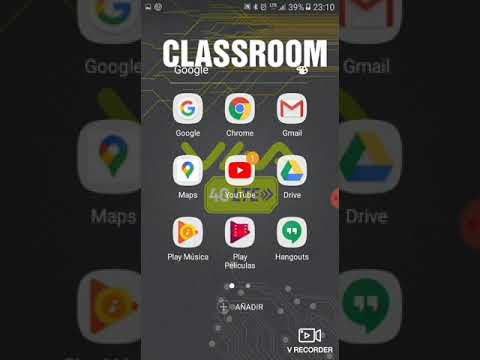This is a detailed screen capture from what appears to be a Google Pixel phone or a similar non-Apple device. The background of the phone displays the word "Classroom" spelled out as "C-L-A-S-S C-L-A-S-S-R-O-M" against a gray backdrop with hints of green. The home screen is populated with a variety of apps. At the top, there are two search apps: "Google Web Search" and "Chrome Web Search." Below those, you can see the "Gmail" app, easily identifiable by its red M icon. Adjacent to Gmail is "Maps," followed by "YouTube," "Drive," and at the bottom, "Play Music," "Play Movies," and "Hangouts." The screen features a color palette including black, dark gray, white, green, with additional accents in red, yellow, and blue. This screen capture gives a glimpse into the main screen of the device, showcasing its organizational setup and color scheme.